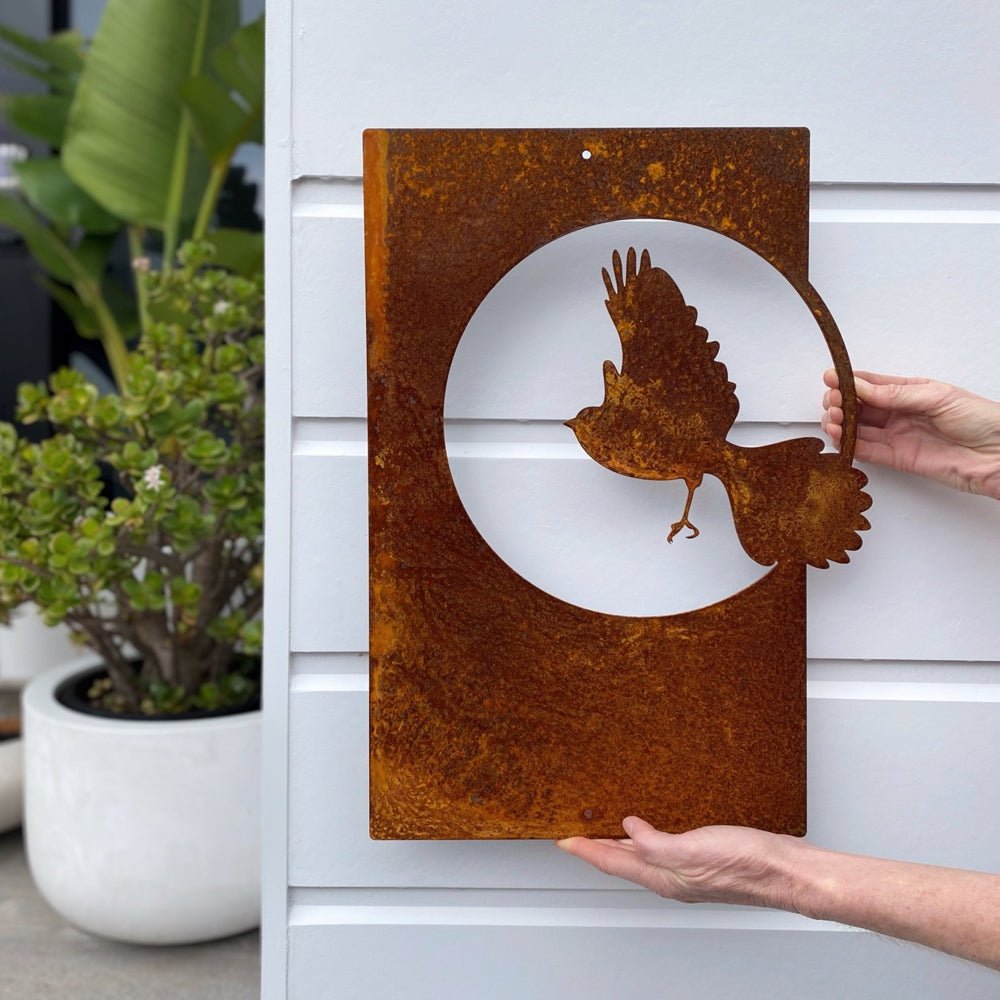Two hands hold up a rusted, bronze rectangular metal artwork outside in daylight. The artwork features a large circular cutout in the center, within which a detailed metal bird is depicted flying, complete with a fan-shaped tail, raised wings, and visible claws on its left leg. The scene includes a white-trimmed wall of a home with plants on the left, some in white planter pots housing succulents and wide-leaf green plants on a gray surface. The hands appear to show how the rusty metal piece, with its intricate bird cutout, would look against the white exterior of the building.